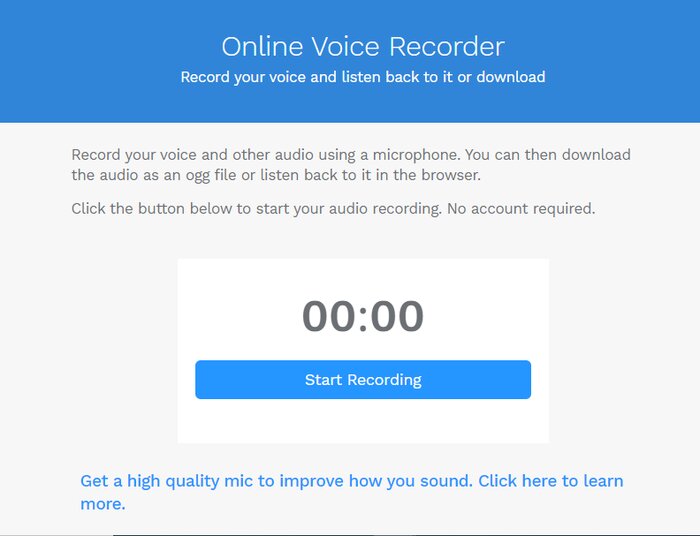The screenshot displays a large square image divided into two main sections. The top quarter features a bright blue background with the text "Online Voice Recorder" in a white bluish color, centered a few lines down from the top. Directly below, also centered, is the text "Record your voice and listen back to it or download."

The remaining three-quarters of the square has a gray background. Approximately a quarter of the way in from the left, in black text, it states, "Record your voice and other audio using a microphone. You can then download the audio as an OGG file or listen back to it in the browser." 

Following a line break, the next line in black reads, "Click the button below to start your audio recording. No account required." Further down and centered is a white rectangle. Near the center of this rectangle are four bolded black zeros, displaying "00:00." 

Below, a bright blue rectangle contains the centered white text "Start Recording." At the bottom, in blue text, it reads, "Get a high-quality mic to improve how you sound. Click here to learn more."